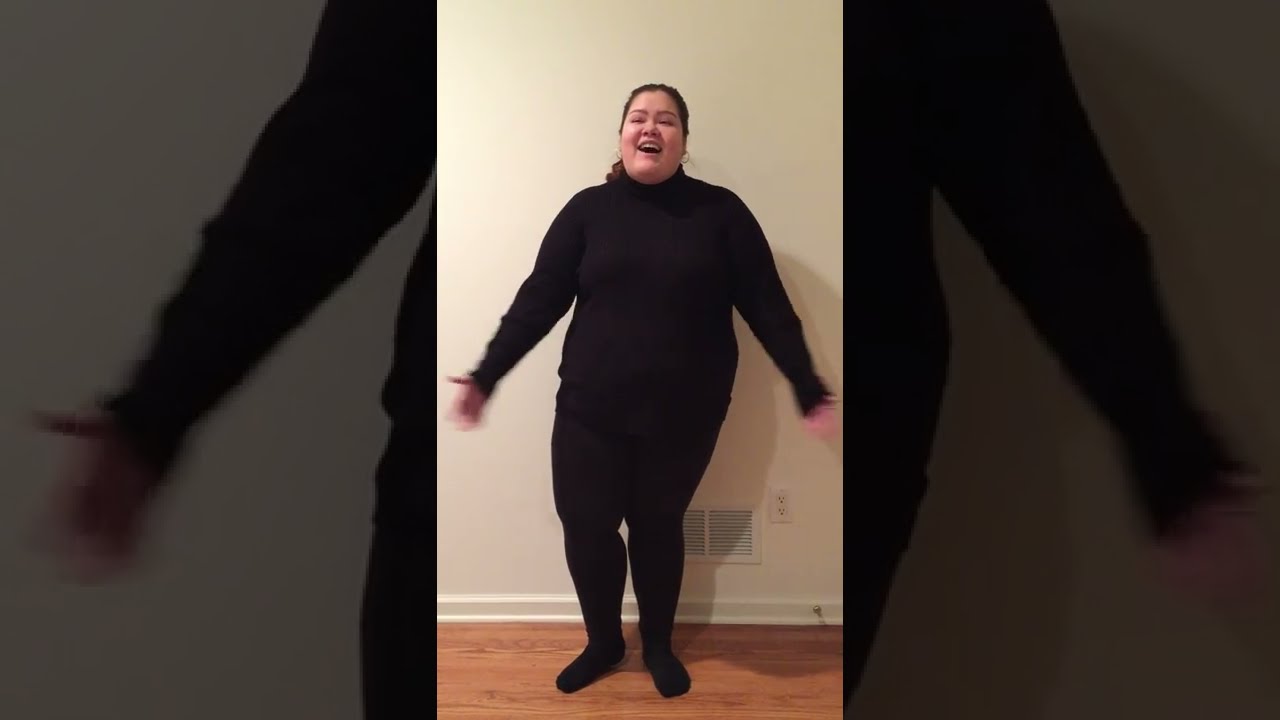The image is a horizontal rectangular photograph with wide black bands on either side and a wider white area in the center, showcasing a woman. She is a young, plus-sized, Latina with dark hair tied in a ponytail, and she is dressed in a black jumpsuit that includes a long-sleeved jacket zipped up to her neck and black pants. Her arms are outstretched, conveying a sense of expression, and her face is animated as if she is talking or singing, with her mouth open in mid-sentence. Behind her is a white wall with a vent at the bottom, along with an electrical outlet. There is also a shadow cast on the wall, indicating that she is leaning against it. The floor beneath her appears to be brown wood or brown tile, though only a small portion is visible. The clipping of the image suggests it might have been taken as a selfie with a smartphone or tablet, similar to a TikTok video format. Notably, her hands are not visible in the frame, and her feet are also outside the photograph's boundaries.